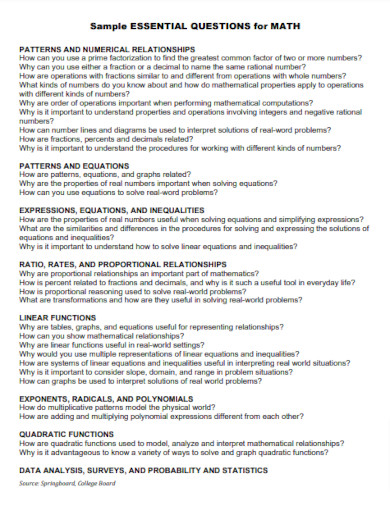The image is a screenshot from a computer or mobile device displaying a document titled "Sample Essential Questions for MATH." The title, prominently located at the top, is in bold with "MATH" fully capitalized. The document is divided into several sections, each addressing different mathematical concepts. 

The first section, labeled "Patterns and Numerical Relationships," begins with the question, "How can you use a prime factorization to find the greatest common factor of two or more numbers?" 

Following this, the section on "Patterns and Equations" asks, "Why can you use either a fraction or a decimal to name the same rational number?" 

The next section, "Expressions, Equations, and Inequalities," includes the question, "How are operations with fractions similar to and different from operations with whole numbers?" 

Under "Ratio, Rates, and Proportional Relationships," a question asks, "What kinds of numbers do you know about, and how do mathematical properties apply to operations with different kinds of numbers?" 

Other significant sections include "Linear Functions," "Exponents, Radicals, and Polynomials," "Quadratic Functions," and finally, "Data Analysis, Surveys, and Probability and Statistics." Each section is similarly detailed with thought-provoking questions designed to explore that specific area of math.

At the bottom of the document, it is credited as a resource from the "SpringBoard College Board."